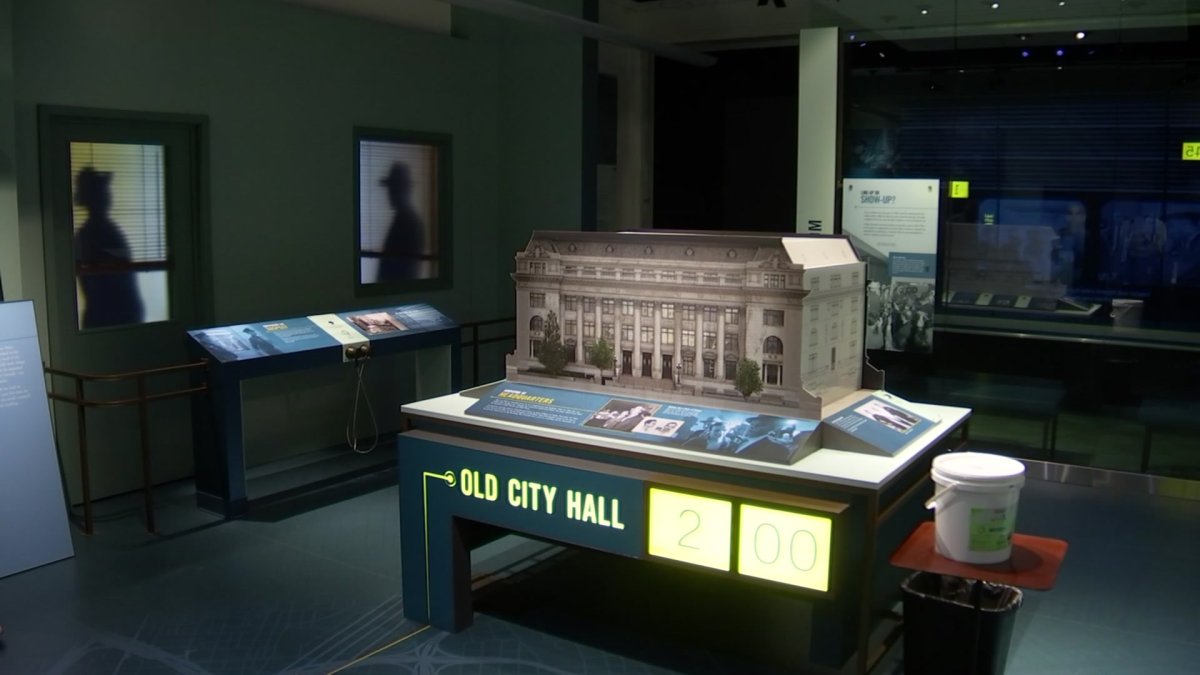The image depicts a detailed, well-lit display likely found in a museum, featuring an elaborate model of a large, three-story, light gray City Hall building with numerous columns and windows, and flanked by small green trees. The model almost fills the rectangular table it sits upon. Text on the table reads "Old City Hall" in yellow against a dark blue background, accompanied by a digital timer showing "2:00" on a bright yellow display. To the right of the model, a small red platform holds a white bucket, possibly filled with spackling, with a black garbage can positioned below. The backdrop includes green walls with glass windows revealing silhouettes of men in hats, a variety of informative posters, and other displays. The overall lighting is dim, except for the model, highlighting its prominence in the presentation.